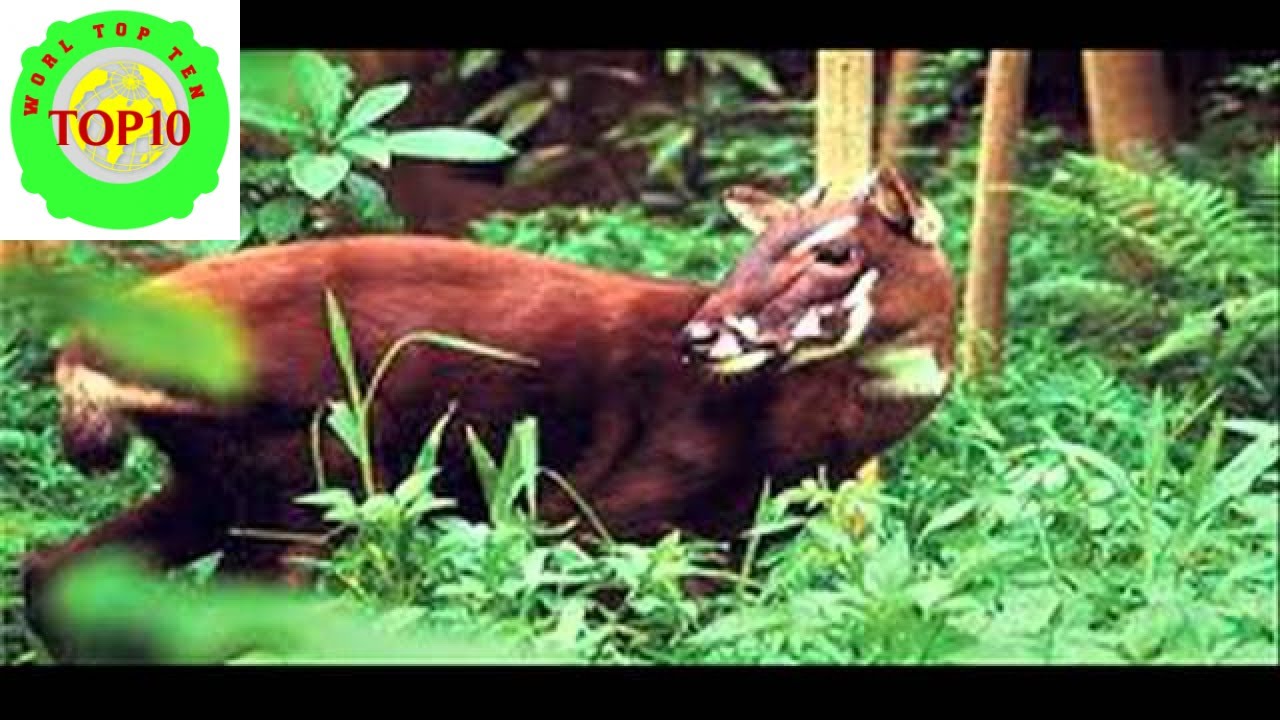The image captures a reddish-brown, deer-like animal with small horns, white facial markings, and a white spot on its chest, set in a lush greenery area filled with ferns, various green plants, and tree stumps. The animal, which also features black and tan coloring, a small tail, and dark fur, is turning its head back, looking towards the left side of the frame. The scene is somewhat blurred around the periphery, especially the foliage in the foreground and sides, adding a sense of depth. Additionally, the photo might be from a show or article, as indicated by the bright green and red symbol in the top left corner, featuring the words "World Top 10," and a yellow cartoon of Earth. The text suggests that the creature is part of a top 10 list, though the context of the ranking is unclear.